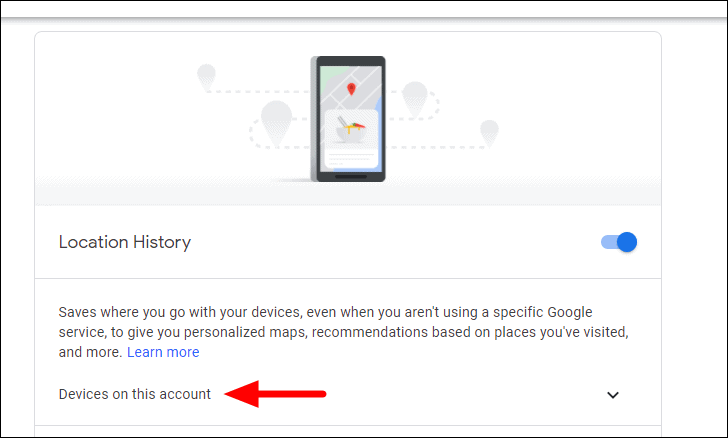In this image, a sleek, designed smartphone occupies the top portion, featuring black outer edges. The screen displays a gray map with a prominent red location icon. This is set against a clean white background that includes four gray icons and a swirling dotted line that curves twice. Below, bold black text reads "Location History," with a toggle switch positioned to the right. The switch is toggled on, indicated by a blue circle.

Beneath this section, a detailed explanation states: "Saves where you go with your devices, even when you aren’t using a specific Google service, to give you personalized maps, recommendations based on places you've visited, and more," followed by a blue "Learn more" link. 

Further down, the text "Devices on this account" appears, highlighted by a red arrow pointing to the left. Adjacent to this is a small box with a downward-pointing arrow inside it. The entire image is framed by a thin black border, maintaining a clean and organized layout.